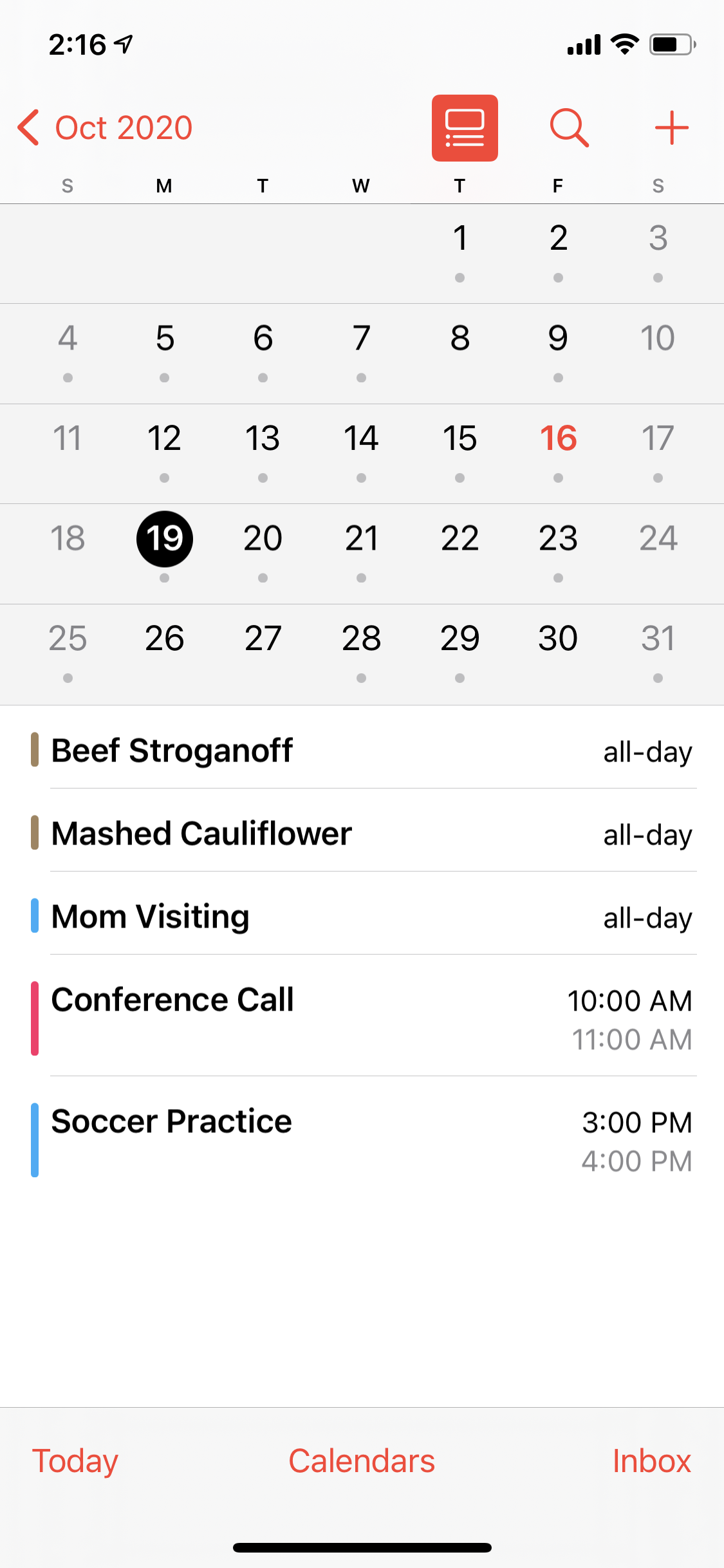The image shows a user's cell phone displaying a detailed calendar with notes. The current time is shown in the upper left corner as 2:16 in black, beside an icon indicating approximately 70% battery life and full signal strength—all set against a light gray background banner that stretches across the top of the screen.

Below this banner, the month and year "October 2020" are displayed in red, accompanied by a back arrow to the left. Toward the right, there's a red box appearing highlighted, containing a white notes icon, followed by a red magnifying glass icon and a red plus sign.

The main calendar occupies the central section of the screen, set against a slightly darker gray background. It starts with Thursday, October 1st, and shows the 19th prominently highlighted with a black circle around it and the number in white, while the other calendar dates are in black. Additionally, the 16th stands out in red, and the dates for Saturdays and Sundays are marked in light gray.

Beneath the calendar grid, several events are listed in bold black letters:
- Beef Stroganoff (all day)
- Mashed Cauliflower (all day)
- Mom Visiting (all day)
- Conference Call (10:00 AM to 11:00 AM)
- Soccer Practice (3:00 PM to 4:00 PM)